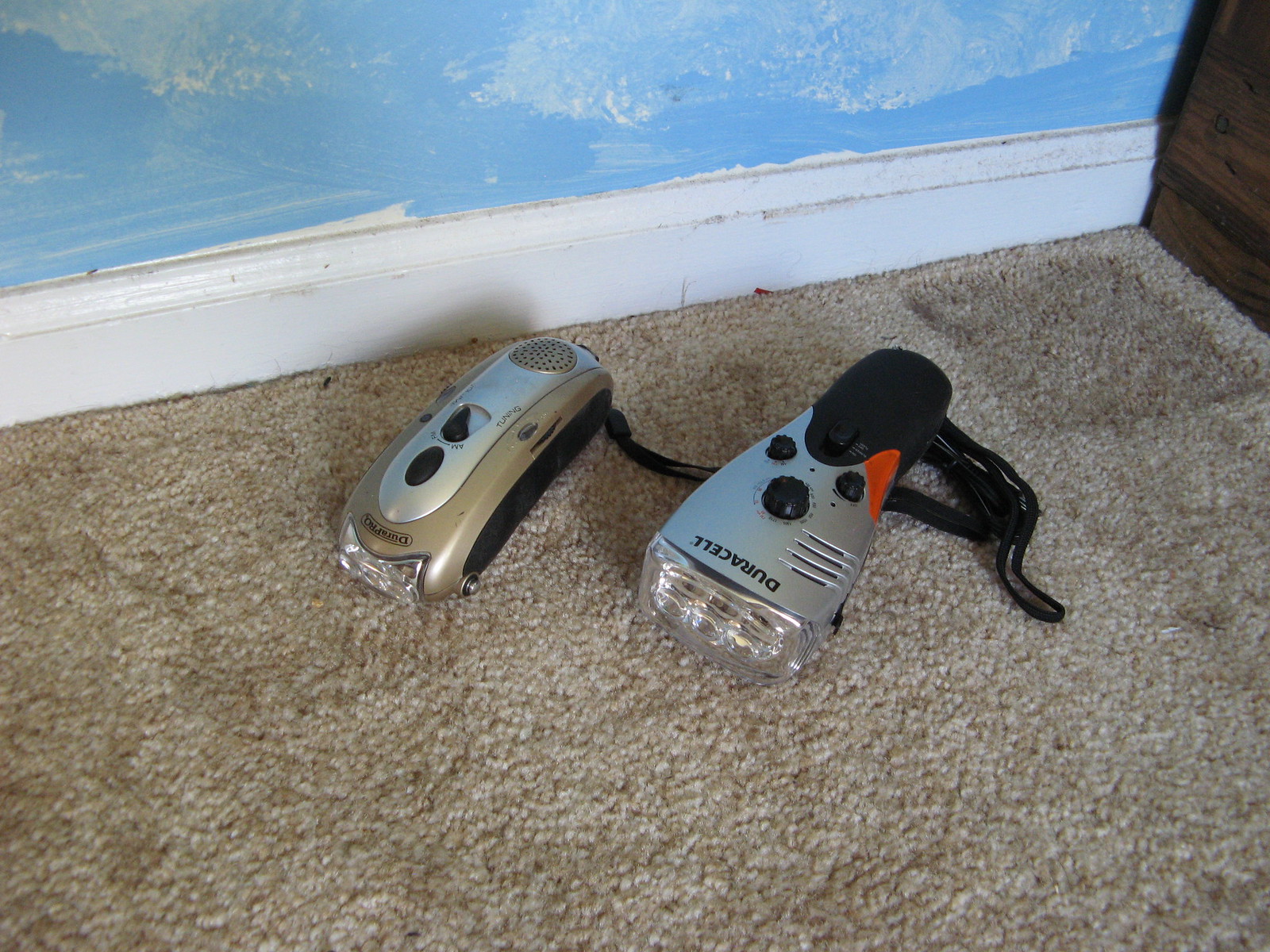The image is a full-color indoor photograph, likely taken in someone's home. The setting features a slightly worn, light brown shag carpet occupying the bottom half of the frame, against which two Duracell-branded radio flashlights are carefully placed. Each flashlight is positioned centrally, with one on the left and the other on the right. Both objects are a mix of tan, gray, black, and a touch of orange. They are equipped with dials, suggesting they might serve as emergency weather radios, and have ropes hanging to the right.

The top half of the image shows a white decorative baseboard that is a bit dirty, above which is a blue wall with white patches showing through, indicating an uneven paint job. In the upper right corner, a small section of dark brown wood is visible, possibly part of a wall or a piece of furniture. The overall impression is a casual snapshot of the two electronic devices arranged on a carpet in a modestly decorated room.